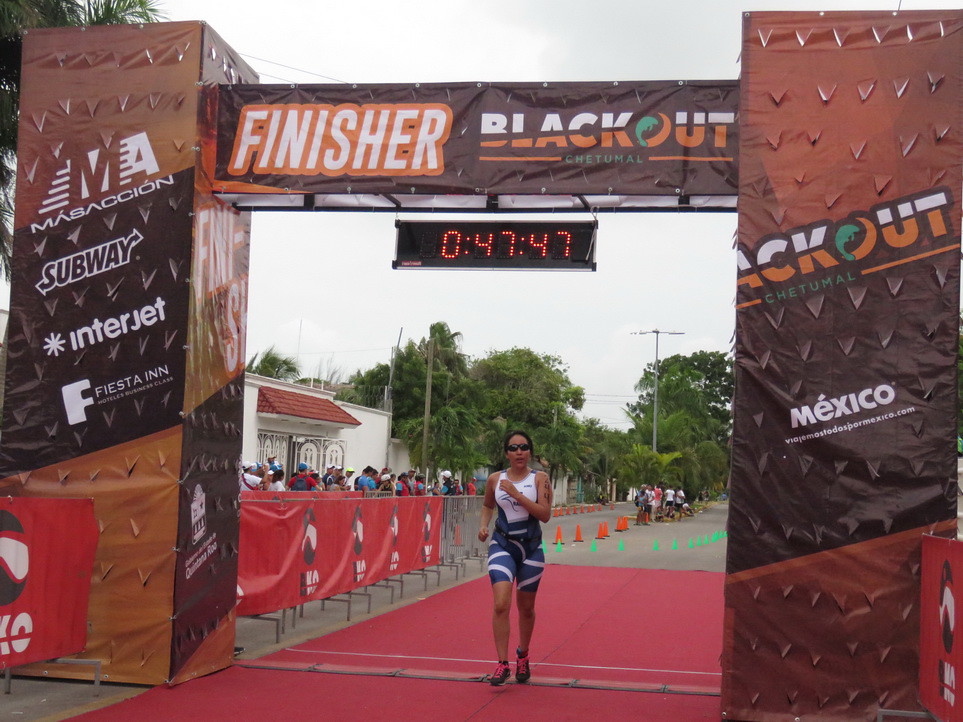The image captures the dramatic conclusion of a race, potentially a marathon, set against the backdrop of vibrant, festive colors. A young woman, wearing tight blue and white shorts, a white sleeveless top, and sunglasses, is crossing the finish line on a red paved area. She also sports a tattoo on her left arm with the number 244, likely her race number. Her shoes are dark with distinctive red or orange laces. Above her, a clock displays a time of 47:47, and a banner with the words "Finisher Blackout" indicates the race name.

The finish line is framed by two pillars adorned in light brown, black, and orange colors, with a white building visible on both sides where spectators are gathered, possibly watching the runner's triumphant moment. The right pillar prominently features the word "Mexico," situating the event in the country, and sponsors' logos like Subway, Interjet, Fiesta Inn, and Mascacion are displayed on the left pillar. Behind the runner, several light green and orange cones are seen, adding to the organized layout, and a fence with red banners that lack any text lines part of the course.